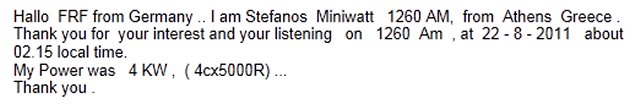In a simple black print on a white background, the text reads: "Halo, FRF from Germany. I am Stephanos Minowot, 1260 AM from Athens, Greece. Thank you for your interest and your listening on 1260 AM at 22-8-2011 about 2:15 local time. My power was 4KW (4CX5000R)." The final line states, "Thank you."